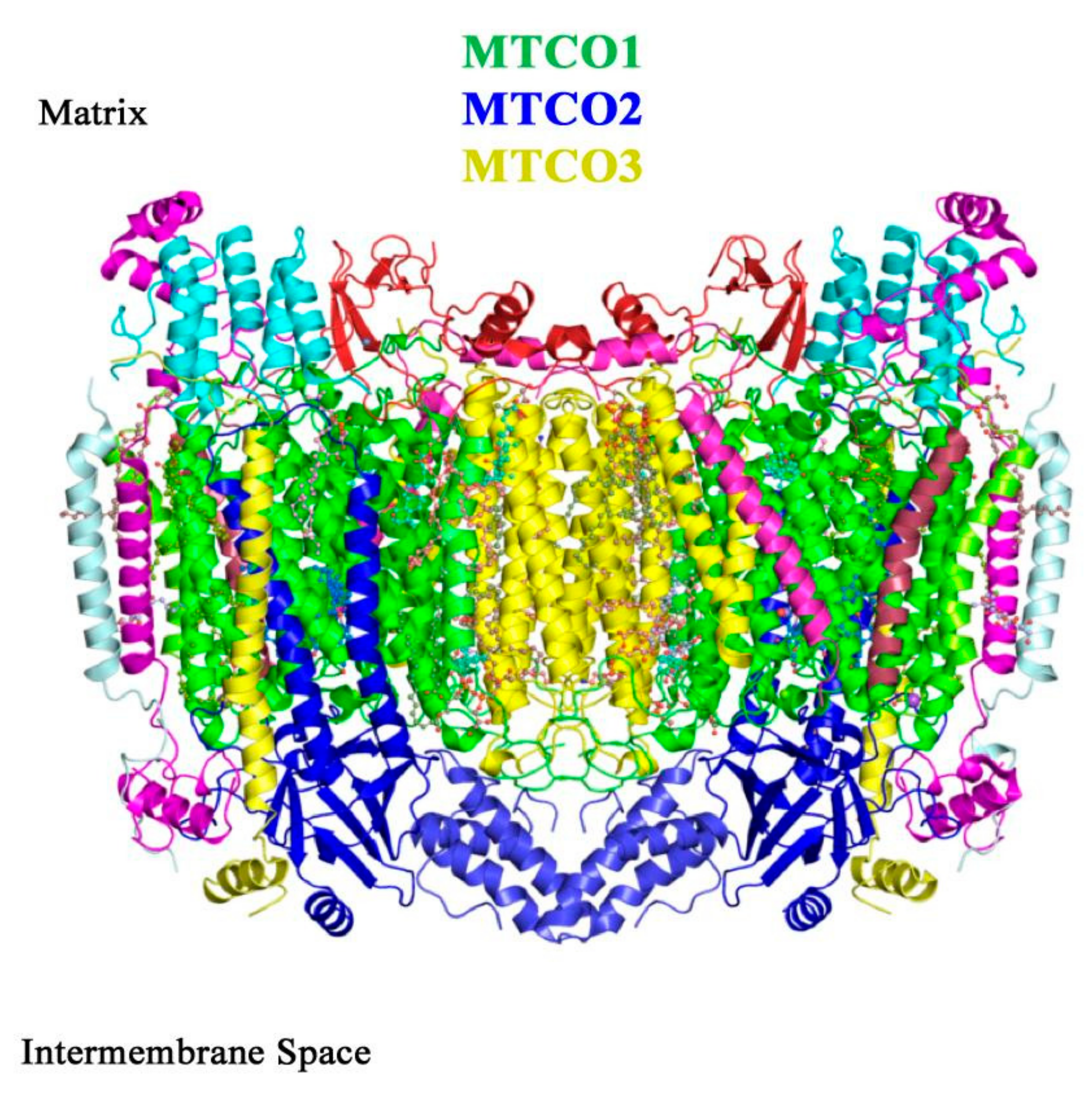This vibrant, colorful image features multiple curly strands resembling ribbons, arranged in a somewhat chaotic yet fascinating pattern against a solid white background, creating a striking visual effect. The composition is devoid of borders, contributing to its floating appearance. These curly strands, which vary in colors including green, yellow, purple, teal, and darker blue, are layered and positioned at different angles. The green strands primarily frame the yellow strands centered in the middle, with some purple appearing more towards the edges and teal and dark blue hues dispersed along the bottom.

Above this central mass of curls, the text "MTC01" (green), "MTC02" (blue), and "MTC03" (yellow) is sequentially listed from top to bottom, lending a structured element to the otherwise dynamic scene. In the upper left corner, the word "matrix" is printed in black text, while "intermembrane space" is noted in the lower left corner, also in black text. Together, these elements merge photographic realism with graphic design and typographic features, creating a diverse and engaging visual landscape.